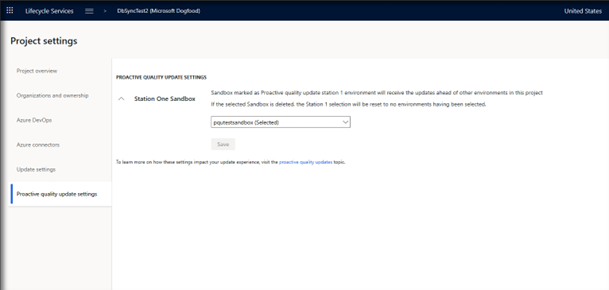The image depicts a blurred screenshot with a predominantly white background. There is a black header at the top of the image. In the upper-left corner, the text "Life Cycle Services" can be discerned. Below this header, there are several navigation elements listed in sequence: "Project Settings," the "Navigation Bar," "Project Overview," "Organizations and Ownership," "Azure Develops," "Azure Correctors," and in bold print, "Proactive Quality Update Settings."

To the right of the "Proactive Quality Update Settings," the text "Station 1 Sandbox" appears, though much of the surrounding text is too blurry to decipher. A notable text block at the bottom right mentions that if the selected sandbox is deleted, the Station 1 selection will be reset such that no environments are selected. The image is quite blurry overall, making some sections difficult to read.